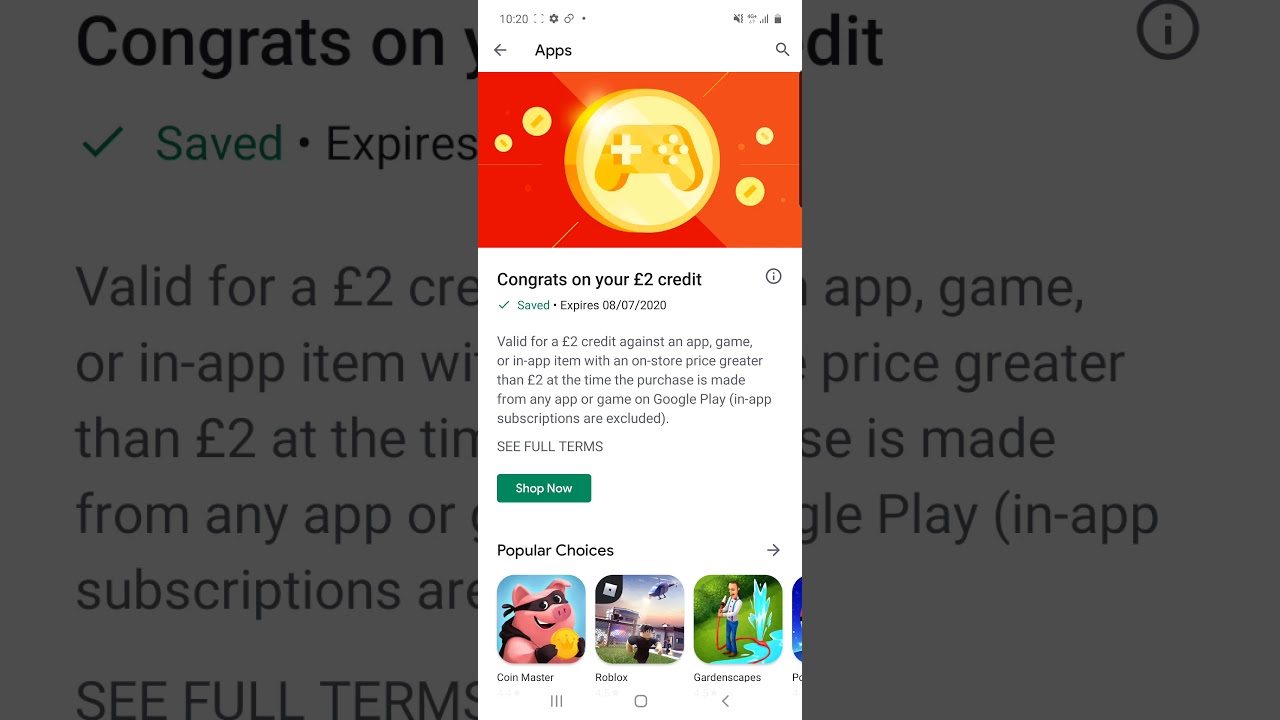This image, sourced from Reddit, features a composite layout where two main elements are layered. The backdrop is a grayed-out Reddit interface, covering about one-third of the image from the left and the last third on the right. Overlaying this backdrop, around one-third from the left, is a smartphone screenshot.

The backdrop displays partial text in the top black bar that reads "congrats on", which gets obscured by the phone screen, reappearing as "DIT" on the right side of the phone. There is a gray circle with an "I" icon, followed by a checkmark and the text "Save . expires", which also partially disappears behind the phone. Beneath this, there are six lines detailing subscription-related information and prices. At the bottom of this section, in bold capital letters, it reads "SEE FULL TERMS".

The phone screenshot includes standard status icons at the top, showing the time, date, Wi-Fi, and battery indicators. Below these, on the left, there's a left-pointing arrow labeled "Apps" with a search icon to the right. Below this top section, there’s a red and light red diagonal stripe along the left side, with a yellow, coin-like symbol in the center featuring a PlayStation controller. This is flanked by two yellow circles on each side. Underneath, in black text, it says "Congrats on your 2 credit euro 2 credit" with a checkmark stating "Saved. Expires 08/08/2070". Following this, there are five lines of information, succeeded by bold text "SEE FULL TERMS". Finally, there is a green tab labeled "Shop Now", under which it says "Popular choices" with three app icons displayed below.

This detailed composition contrasts the grayed Reddit layout with the vibrant smartphone screenshot, encapsulating a mix of celebratory prompts, subscription details, and app suggestions.